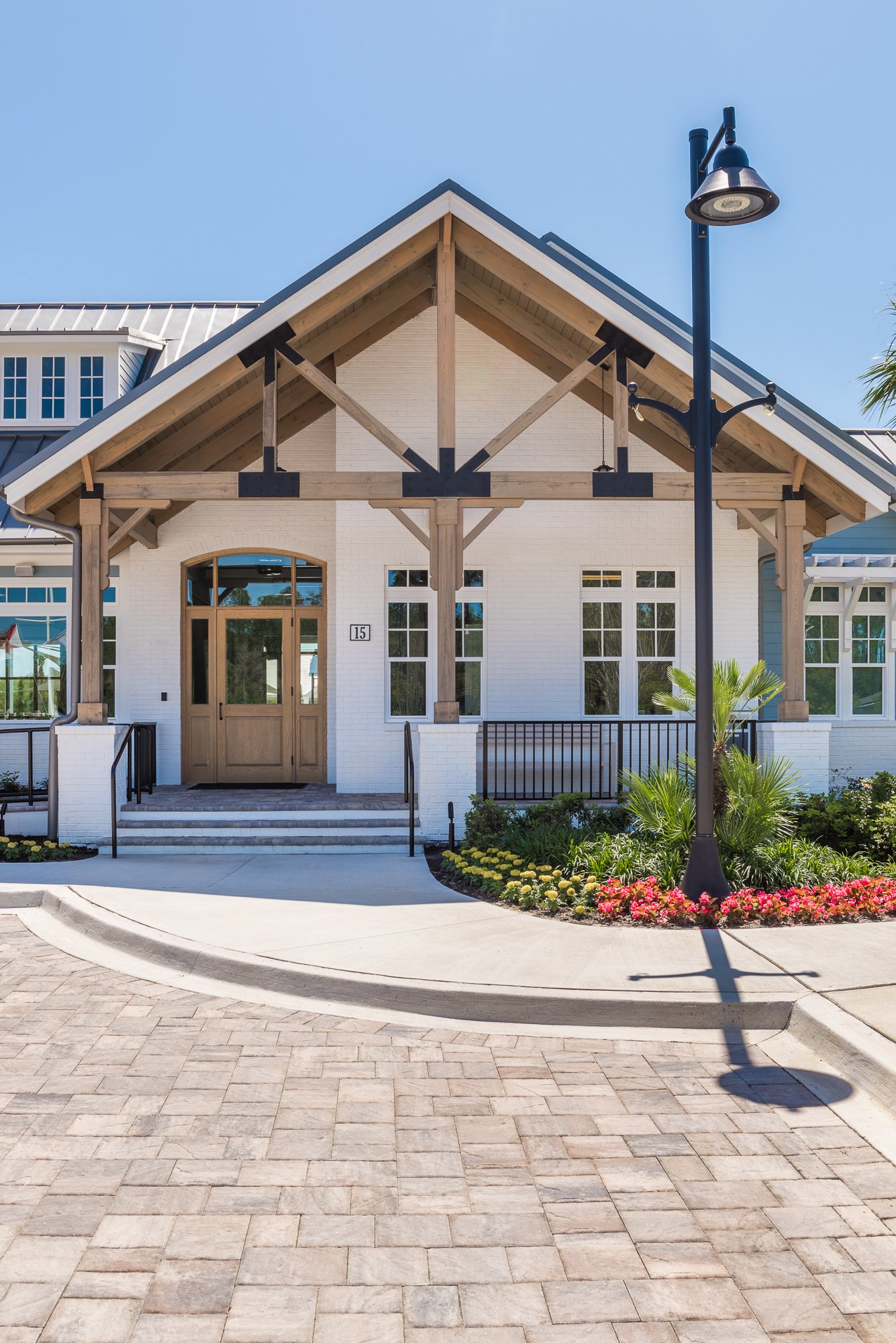In this photograph, captured in portrait view with a vibrant, cloudless blue sky as the backdrop, the focal point is a charming white house numbered 15. It features a prominent upside-down V-shaped roof with intricate wooden rafters. The house has a large wooden door, complemented by substantial windows alongside. Leading up to the door are three steps, flanked by black railings. In front of the house, a brick-paved area and a beautifully landscaped garden with yellow and red flowers, small shrubs, and a circle of plants add to its appeal. A tall black lantern-style light, situated by the walkway, and a glimpse of another two-story white-roofed building in the background, complete the picturesque scene.